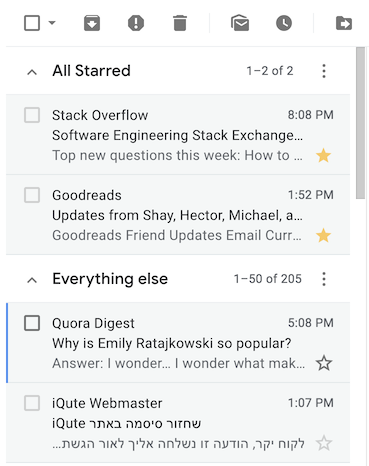This image captures a screenshot set against a white background, focusing on a structured interface with various icons and text.

At the top header, there are multiple icons arranged from left to right:
- The first icon is a small black square containing a white arrow pointing downwards.
- This is followed by an exclamation point inside a black octagon.
- Next to it, there's a trash can icon.
- Following the trash can is a letter icon.
- Nearby, there's a clock icon displayed in bold black text.
- Right beside it, all starred items are indicated.

To the right of these icons, gray text reads "1 to 2 of 2". Beneath this header, larger text states "Stack Overflow - Software Engineering Stack Exchange," timestamped at "8:08 p.m."

Below this section, there is an update from Goodreads:
- It shows update information from "Shea Hector Michael."
- The subject line indicates a Goodreads friend update email.
- The time is marked at "1:52 p.m."
- There is a yellow star positioned to the lower right of this content.

Further down, in bold black text, the interface reads "Everything Else 1 through 50 of 205."